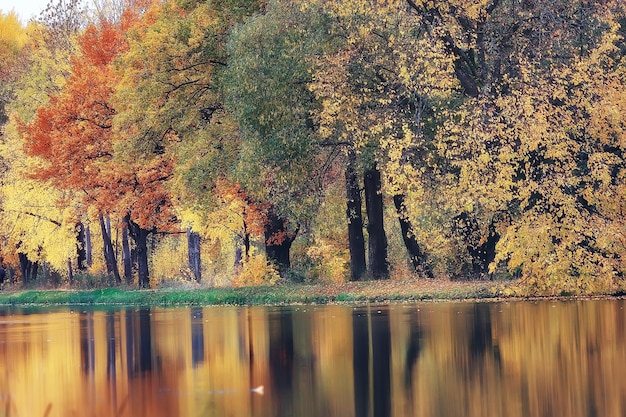This image depicts a breathtaking fall landscape centered on a serene pond that mirrors the vibrant array of trees above it. Dominated by the rich and varied hues of autumn, the scene begins on the left with golden leaves, transitions through deeper oranges and greens, and culminates on the right with a bushy tree adorned in bright yellow foliage. The trees, characterized by their height and dotted leaves suggestive of fine brush strokes, span across the entire backdrop and foreground, creating a golden hue throughout the photograph. A narrow strip of lush green land precedes the still water of the pond, amplifying the reflection of the vividly changing leaves under the clear, sunny sky. No people are present, allowing the natural beauty of the landscape to occupy the viewer's undivided attention.